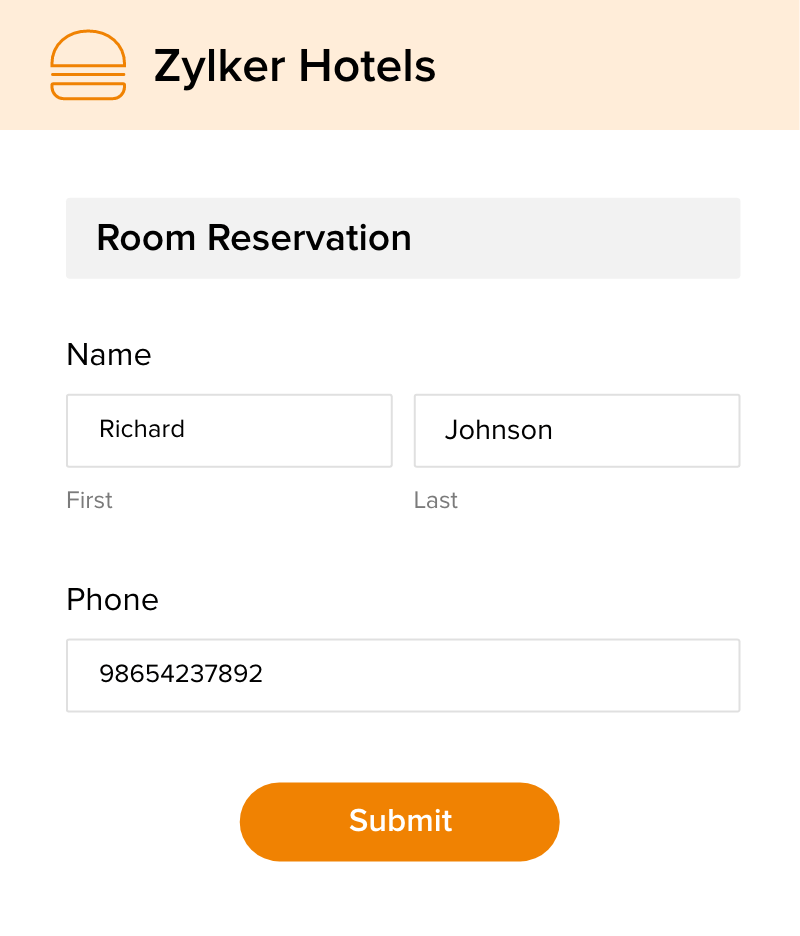The image is a screenshot from Zylker Hotels, spelled "Z-Y-L-K-E-R". In the top left corner, a minimalistic hamburger icon is displayed, featuring a top and bottom bun with an orange line in between symbolizing the patty. The background of the interface is a light flesh tone. Beneath this, the design transitions to a predominantly white background with a grayish rectangular box labeled "Room Reservation."

Within this box, there are input fields for user information. The fields for the first and last names display "Richard" and "Johnson" respectively. Below the name fields is another white rectangular input area labeled "Phone," showing the phone number 986-542-37892.

At the bottom of the screenshot, an eye-catching orange pill-shaped button with a white font is prominently positioned, marked "Submit." The layout is suggestive of a simple and clean user interface, potentially part of either a desktop or mobile application.